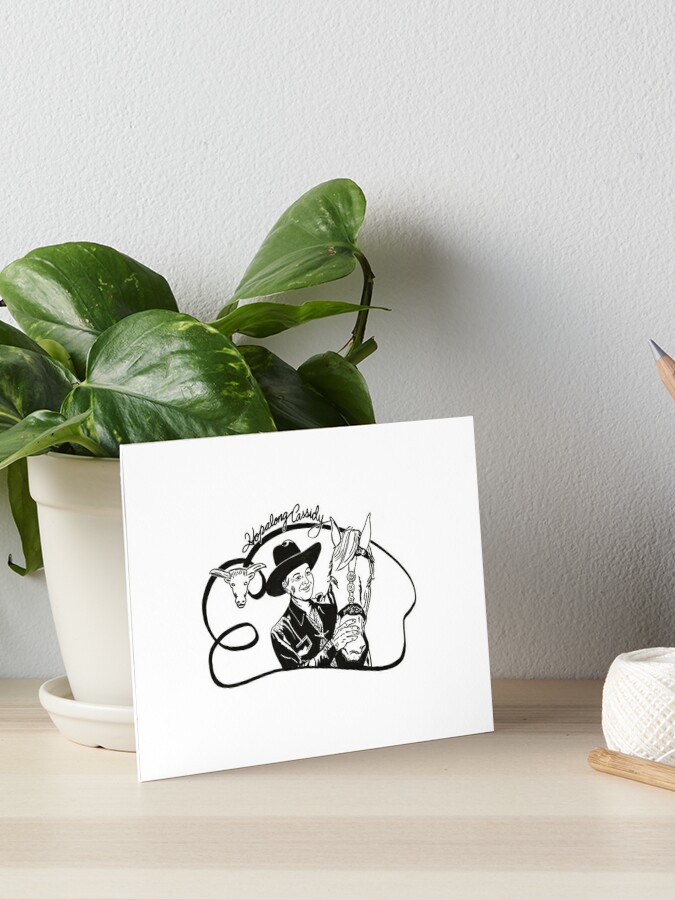This photograph captures a beautifully detailed arrangement featuring a greeting card of sorts, prominently displayed against a potted plant backdrop. The card, portraying an illustration of a cowboy petting the head of a horse, features the text "Hop Along Cassidy" in an intriguing, almost signature-like font. The illustration, rendered in black ink, shows the cowboy in a black hat and collared jacket, with the horse's head depicted facing the viewer. The image is enclosed by a wavy, swirling outline that adds a dynamic touch.

The card is rectangular and set at an angle against a houseplant in a white pot. The plant, standing about 12 inches tall, has large, lush green leaves that drape gracefully over the pot. The pot itself is simple, with rims on the top and bottom, and rests on a light brown wooden tabletop. 

To the right of the composition, a ball of white string or yarn adds a subtle detail, along with a partially visible pencil. The background is a white wall, imbued with delicate shadows cast by the plant and the card, enhancing the photograph's depth and texture. The overall setting is serene yet detailed, blending the elements together in a harmonious tableau.